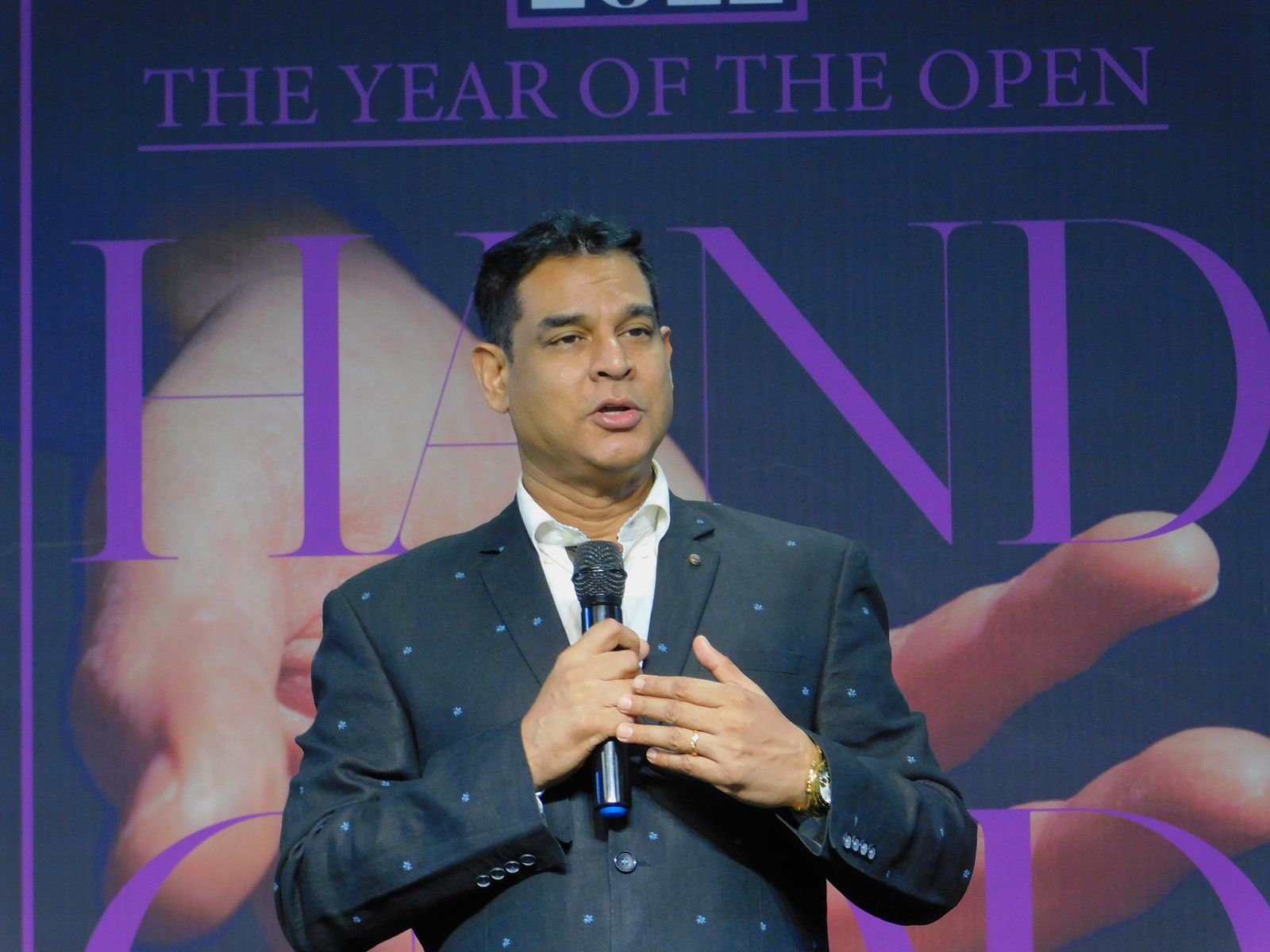The image depicts a man with light brown, olive-toned skin and short black hair, standing from the waist up in front of an audience, possibly giving a talk or speech, or appearing on television. He is dressed in a dark gray suit jacket adorned with blue embroidered dots, paired with a white collared shirt. The man is engaged in speaking, evidenced by his open mouth, and he holds a microphone in his right hand. On his left hand, he wears a gold wedding ring and a gold watch. The backdrop behind him prominently features the phrase "The Year of the Open" in purple, with the word "Hand" and an image of an open hand, suggesting it may be the title of his speech or the event theme, potentially a TED Talk or a convention.